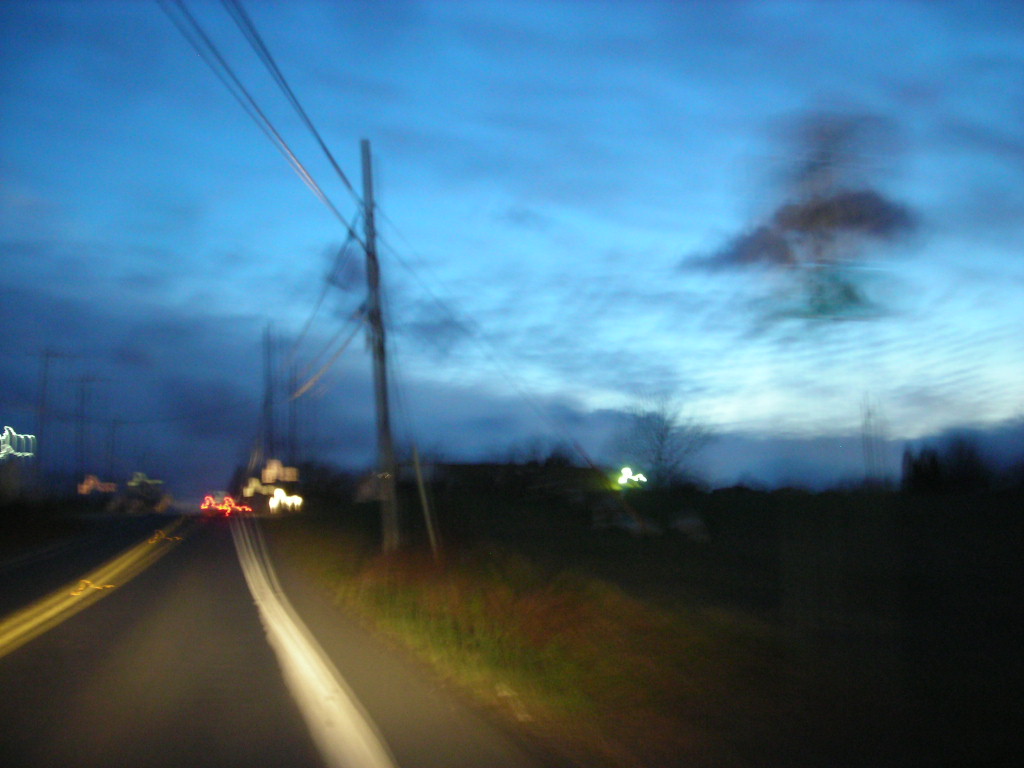A blurry photo taken at dusk portrays a highway scene under a medium blue sky scattered with clouds. The horizon shows mountains, darker and more prominent towards the left and gradually descending towards the right. The setting sun creates a gradient of whiter blue near the horizon. A peculiar dark smudge, resembling a head with arms and legs, is seen against the sky. On the left side of the image, a two-lane highway stretches with a yellow center line and white outer lines. In the distant background, neon lights—some featuring red cursive writing and white illumination—add a hint of human presence. The right side of the road is flanked by grass, telephone poles, and an open field.